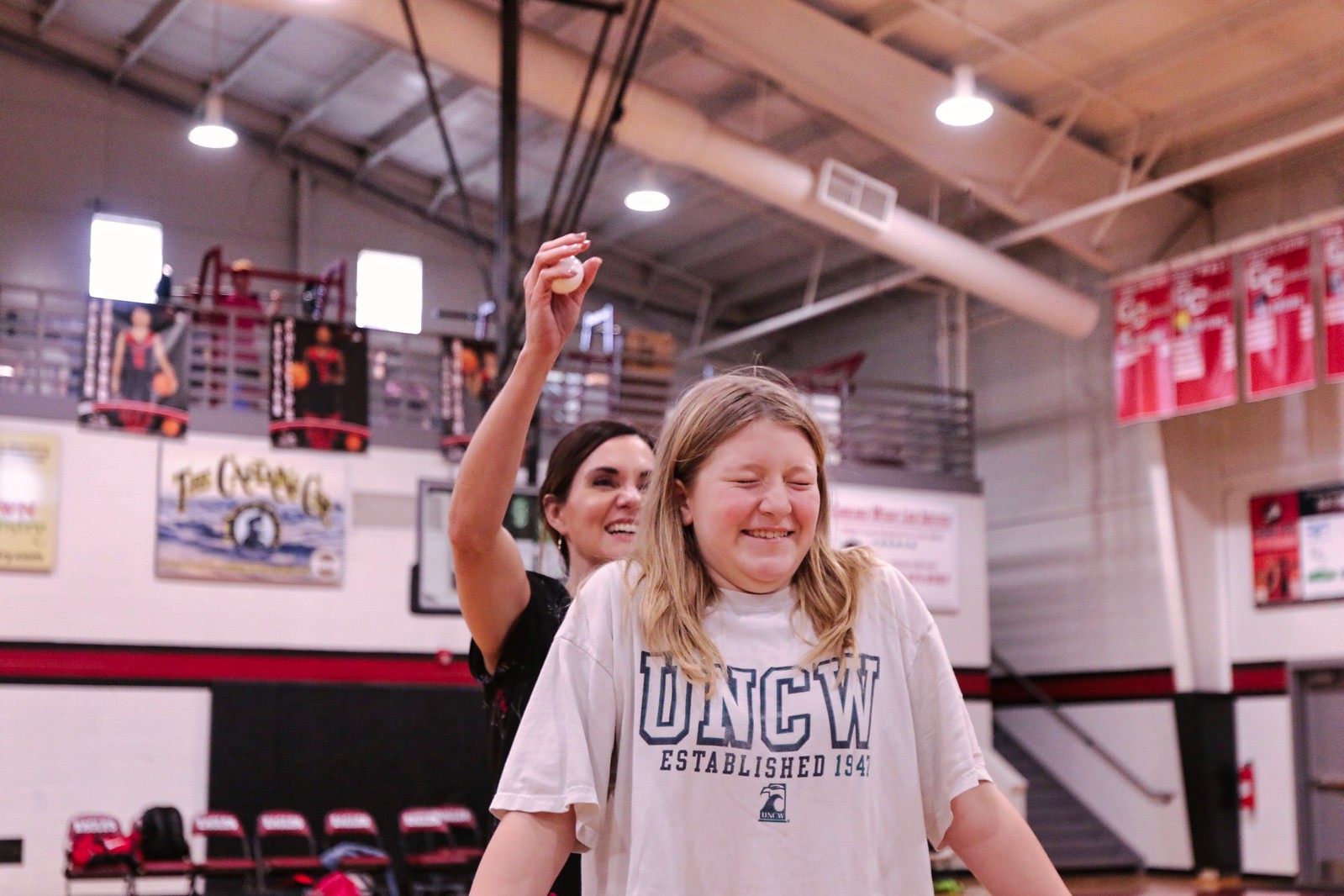The photograph captures a lively scene inside a school gymnasium adorned with red and white colors, hinting at the school's theme. The gym features high ceilings, incomplete with hanging lights, surrounded by banners and posters of basketball players and various achievements. Folded chairs and stairs leading to potential bleachers can also be seen.

Central to the image are two women - a younger girl, possibly a teenager with dirty blonde hair, and an older woman with brown hair tied back. The girl is wearing a large off-white t-shirt reading "UNCW, established 1947," and stands with her eyes shut tight, her shoulders scrunched up, bracing for some anticipated impact. Behind her, the older woman, dressed in a black blouse, smiles in amusement and holds a white object resembling either a ping-pong ball or an egg above the young girl's head, suggesting that an experiment or a playful moment is about to unfold.